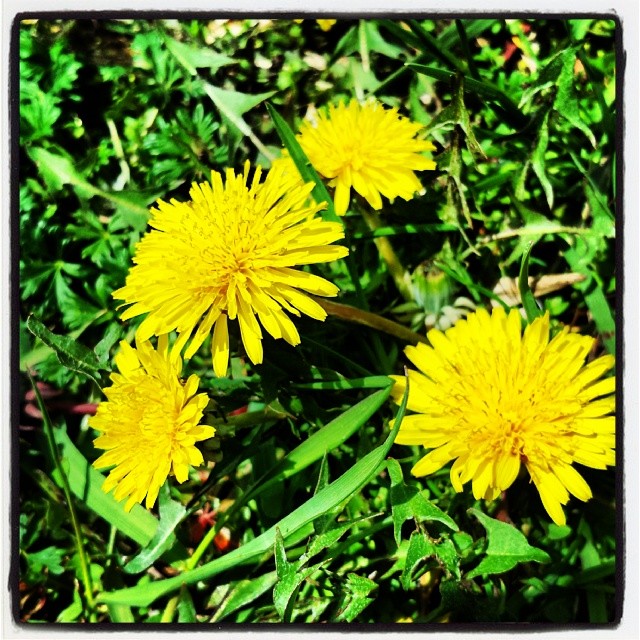This detailed, square-format color photograph captures a group of four dandelions in full bloom amidst a background of densely packed green vegetation, showcasing a mix of regular-sized and long, thin leaves. Each dandelion blooms with a deeply golden color, its flower heads densely covered in many florets. The stems, visible in parts, exhibit a reddish hue adding contrast to the green surroundings. Notably, the layout places three dandelions toward the left side—comprising a larger flower in the center flanked by two smaller ones—and a much larger, fully open dandelion toward the bottom right. Sunlight casts subtle shadows behind the blossoms, accentuating their prime condition on this sunny day. Buds hint at more blooms to come, adding potential life to this vibrant, realistic capture.